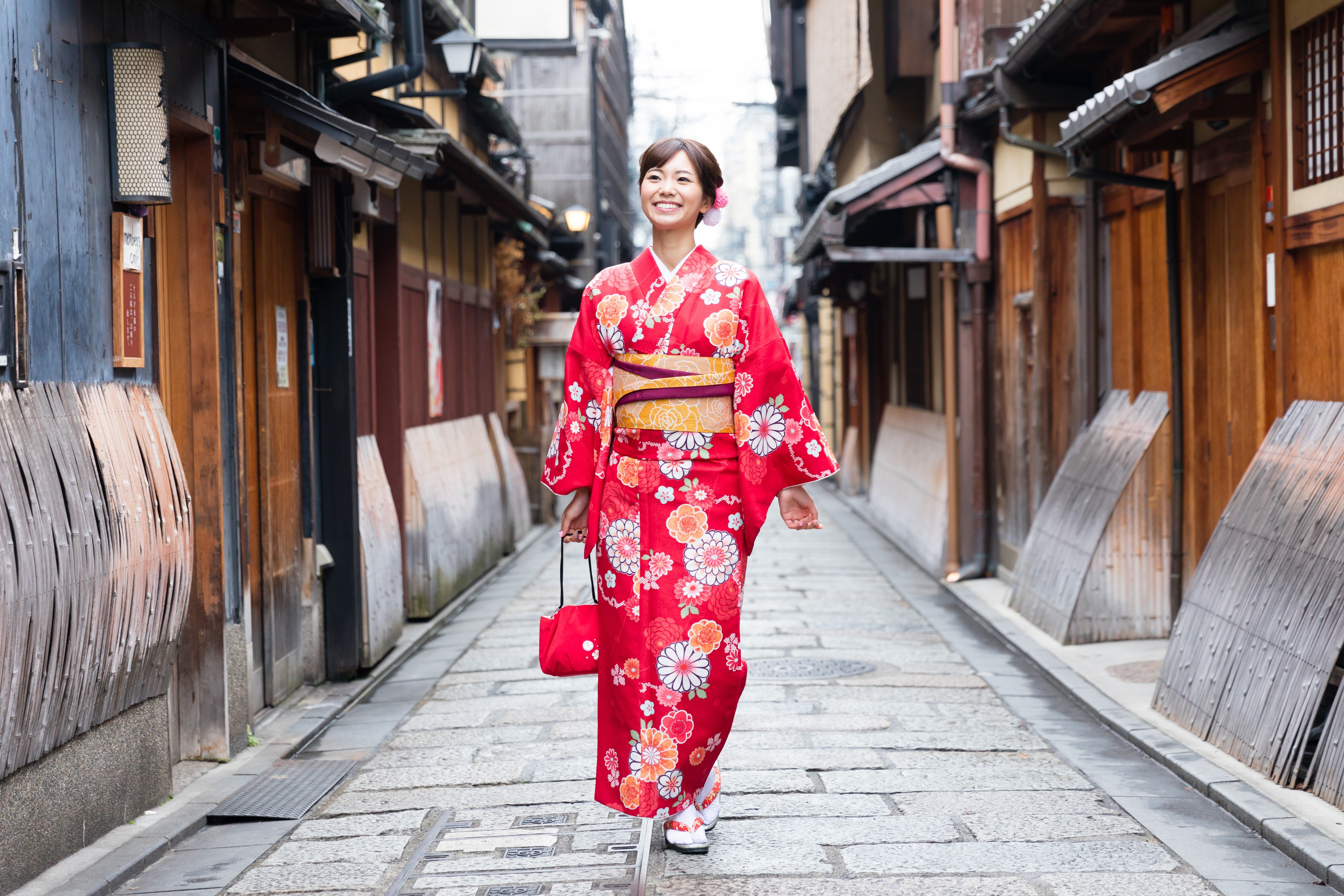This picture captures a joyful Asian woman walking down a narrow, cobblestone street in what appears to be a Japanese city. The street is framed by wooden buildings on both sides, some adorned with wood paneling and straw-like structures. The woman, dressed in a striking red kimono adorned with a variety of colorful flowers in shades of white, orange, pink, and dark pink, smiles brightly as she walks towards the viewer. Her ensemble is completed by a yellow and burgundy waistband and red sandals worn over white socks. She carries a small, dark red purse with white dots in her right hand and has two pom-poms—a pink and a white one—decorating her hair. The overall scene evokes a sense of traditional charm and vibrant happiness.